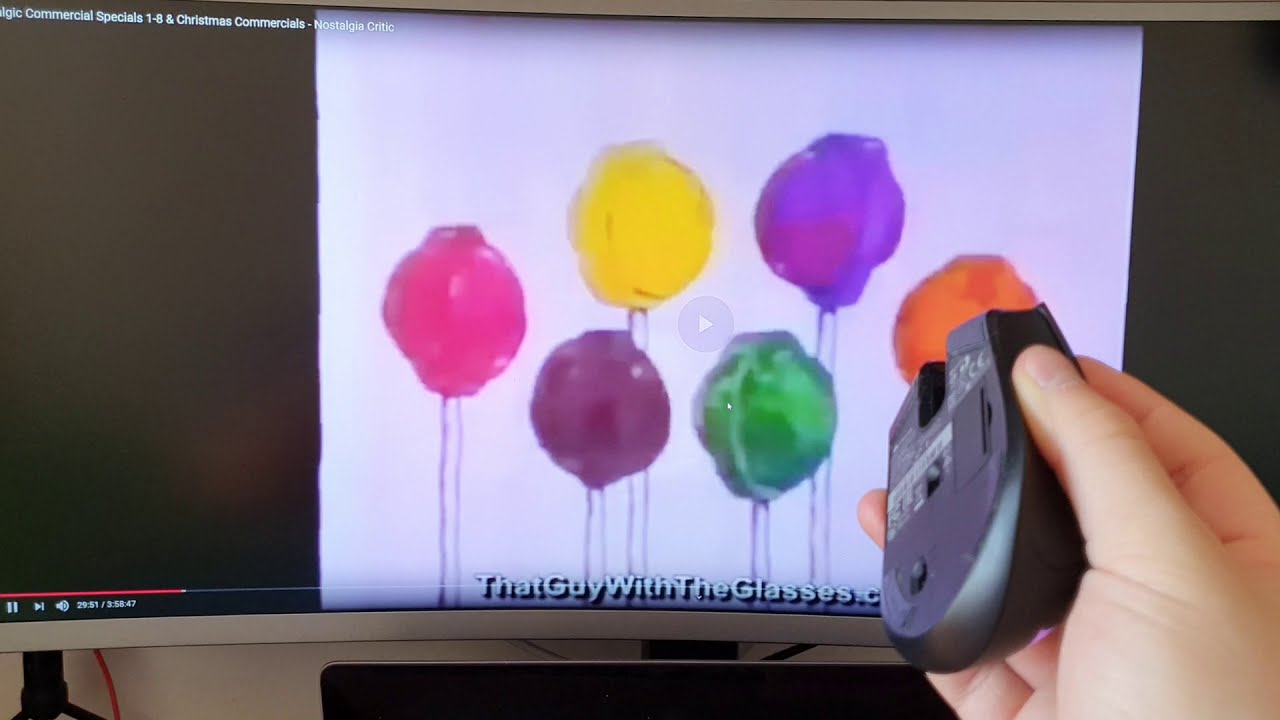The image depicts a photo of a wide, possibly curved, computer monitor or television screen displaying a paused YouTube video. The screen features a white background with six lollipops painted in vibrant watercolor shades, from the left to right: pink, yellow, purple, orange, dark plum purple, and green. These lollipops are round with ridges and are mounted on clear sticks. Above the lollipops, text in white reads, "Commercial Specials 1-8 and Christmas Commercials - Nostalgia Critic."

In the bottom portion of the screen, another white text with black shadowing says, "That Guy With The Glasses." On the lower left, there is a red progress bar indicating the video’s play position, paused at 29 minutes and 51 seconds of a total duration of 3 hours, 58 minutes, and 47 seconds. The screen also features playback controls, including pause, play, next, and a speaker icon, on a black bar beneath the video.

In the lower right corner of the image, a Caucasian hand is holding up a wireless computer mouse, showcasing its underside. The mouse is dark gray, with the thumb positioned on top, gripping it securely. The left section of the screen is predominantly black, indicating either a blank area or a part of the video that hasn't loaded.